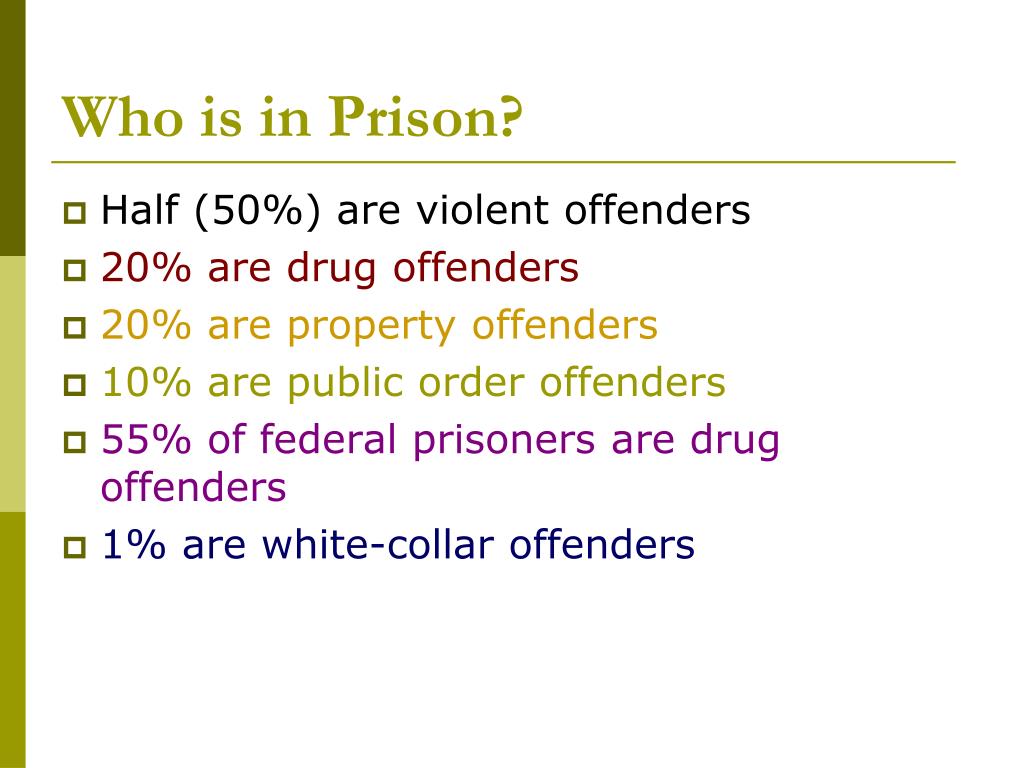This image is a cropped snapshot of a white-background informational slide or document titled "Who is in Prison?" It features a thin vertical green stripe on the left side in three shades of green, and a very thin green line under the title. The slide contains six bullet points, detailing the percentages of different types of offenders, each marked with square bullets. The bullet points are as follows:

- 50% are violent offenders
- 20% are drug offenders
- 20% are property offenders
- 10% are public order offenders
- 55% of federal prisoners are drug offenders
- 1% are white-collar offenders